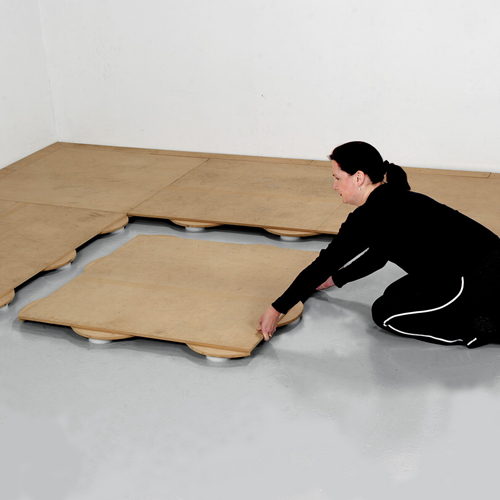In this indoor photograph, an older woman with dark black hair, tied back in a ponytail, is seen kneeling on a gray cement floor, resting on her shins and forearms. She is dressed in a black tracksuit with a white stripe along the sides and is wearing an earring. The woman is meticulously aligning a beige wooden tile, pushing it with the palms of her hands to fit snugly against previously placed tiles. The tiles, each supported by circular disc-like feet, suggest they are part of a modular flooring system. A single row of three tiles is already in place, and she is adding a fourth tile to the second row. The setting is a plain, bare room with a white backdrop, highlighting the minimalist and focused nature of her task.